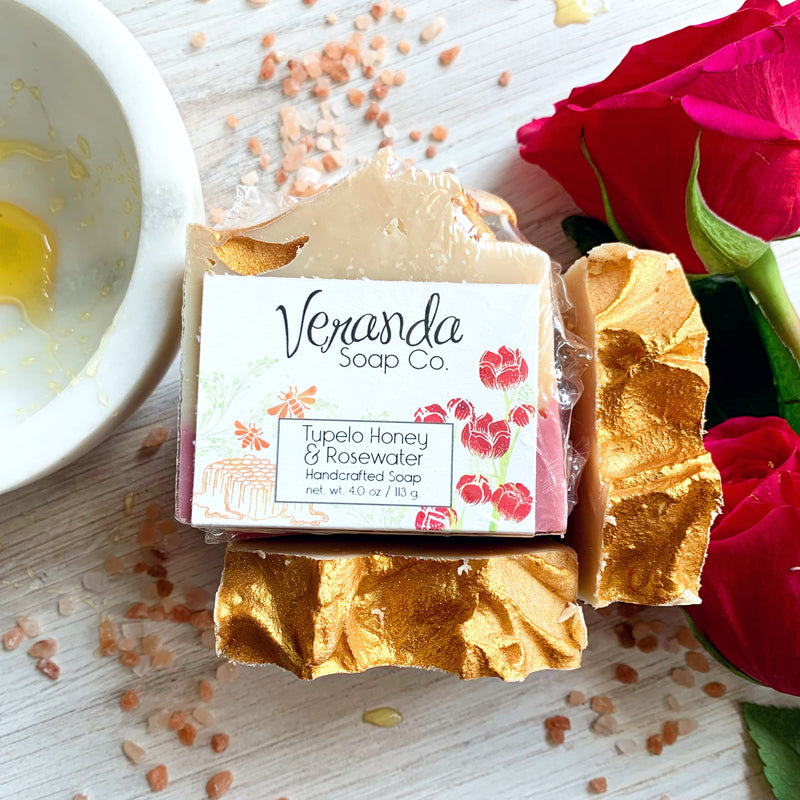A detailed photograph of handmade Veranda Soap Co. soap bars displayed on a whitewashed wood grain table. The centerpiece is a bar of Tupelo Honey and Rosewater Handcrafted Soap, wrapped in plastic, emblazoned with the company name in cursive, two bees above a honeycomb, and red flowers with pale green stems. The soap weighs four ounces (113 grams). Uneven, scalloped edges give it an artisanal look. Surrounding the central soap is another bar beneath it and one to its right, with two half-opened red rosebuds nearby, their green stems visible. Sprinkled on the table are what appear to be large grains of Himalayan salt in shades of orange, white, and pinkish hues. To the left of the soap, partially cut off, is a marble bowl with a small amount of yellow liquid. The wood grain of the table runs diagonally from the upper right to the bottom left.